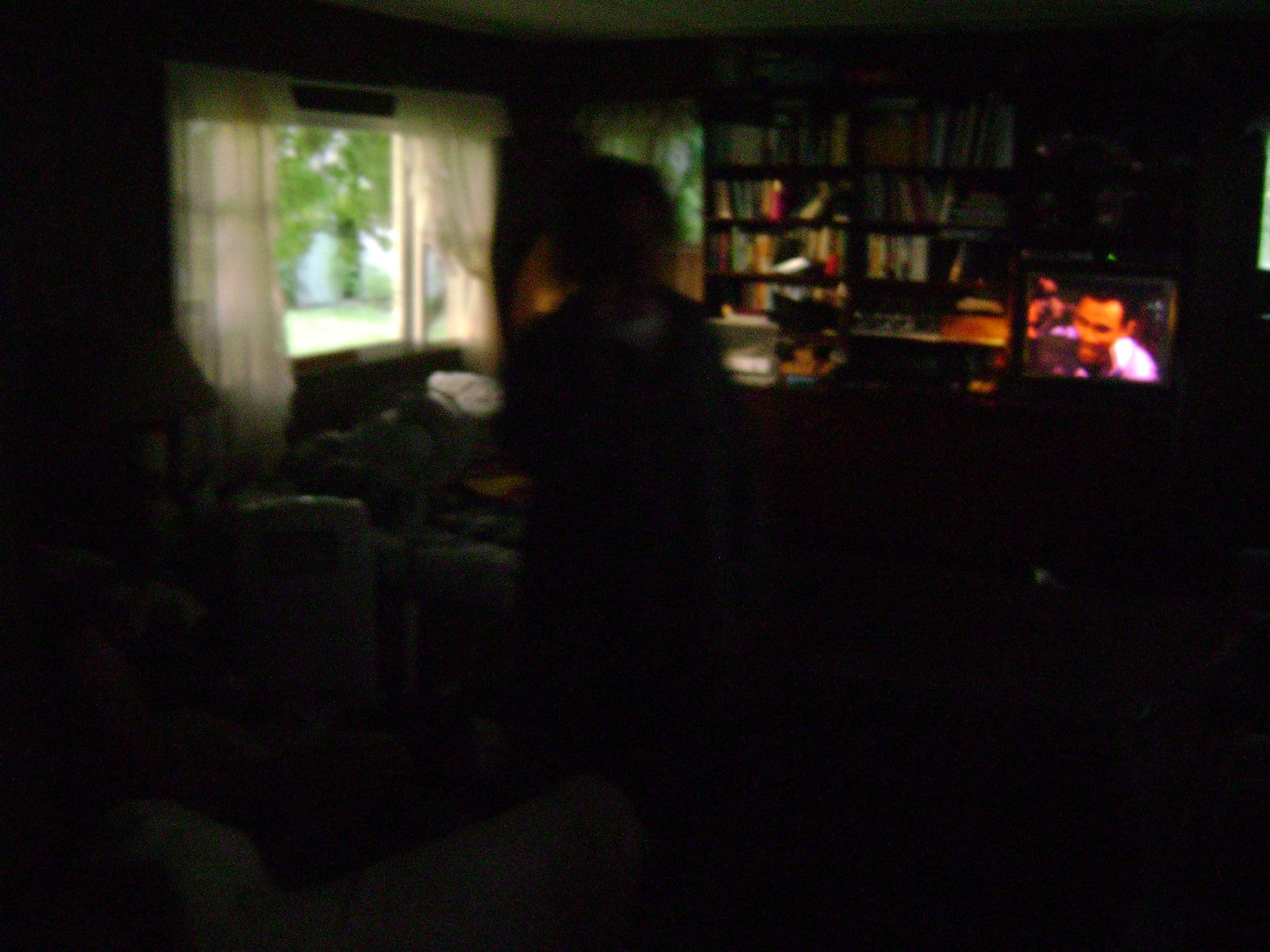In this dimly lit room, the left side of the image features a window with the curtains pulled back, revealing an outdoor scene with a tree visible through the glass. The room is otherwise enveloped in darkness. On the far wall, there's a framed picture hanging, and two well-stocked bookcases brimming with books stand prominently. A desk can be spotted in the shadowy space, upon which sits a tablet or computer displaying a picture of a man. A faintly discernible person is present in the scene, but the lack of light obscures their details. Nearby, there is either a couch or a bed cluttered with various items. The overall image appears to be slightly blurred, adding to the mysterious ambiance of the setting.